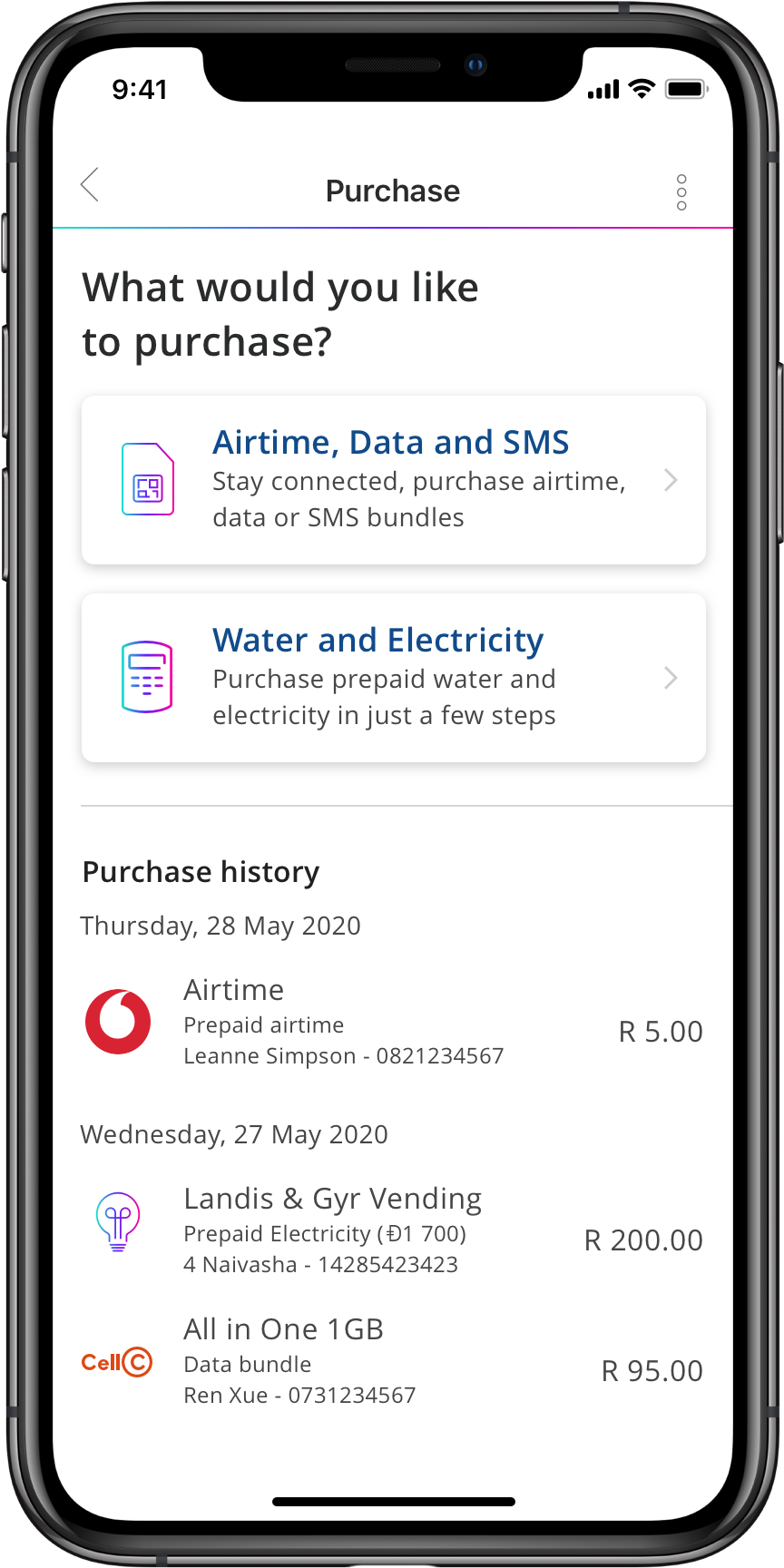The image depicts a highly detailed illustration of a smartphone, shown almost at actual size. The level of detail is so precise that one can distinctly make out the side controls of the phone. At the top of the screen, the status indicators display: the time (9:41 AM), signal strength, Wi-Fi signal strength, and a fully charged battery icon.

Central to the screen, beneath these indicators, is a heading labeled "Purchase," underlined by a fine gradient line that transitions from light blue on the left, through purple, to pink on the right. Below this heading, a large question reads, “What would you like to purchase?” 

Under this question, two bordered panels are displayed. The first panel reads "Airtime, Data, and SMS" in dark blue font, with a subtext that says, "Stay connected: Purchase airtime, data, or SMS bundles." The second panel, labeled "Water and Electricity" in blue font, is accompanied by the subtext, "Purchase pre-paid water and electricity in just a few steps."

A fine gray line separates these panels from the lower half of the screen, which displays a purchase history. This section lists:

- On Thursday, May 20, 2020, the purchase of airtime priced at 5 R (currency not specified).
- On Wednesday, May 27, 2020, two purchases: "Landrus and Jir bending" at R200 and an "All-in-One 1GB data bundle" at R95.

This comprehensive depiction serves as both a visual guide and a detailed record of recent transactions.